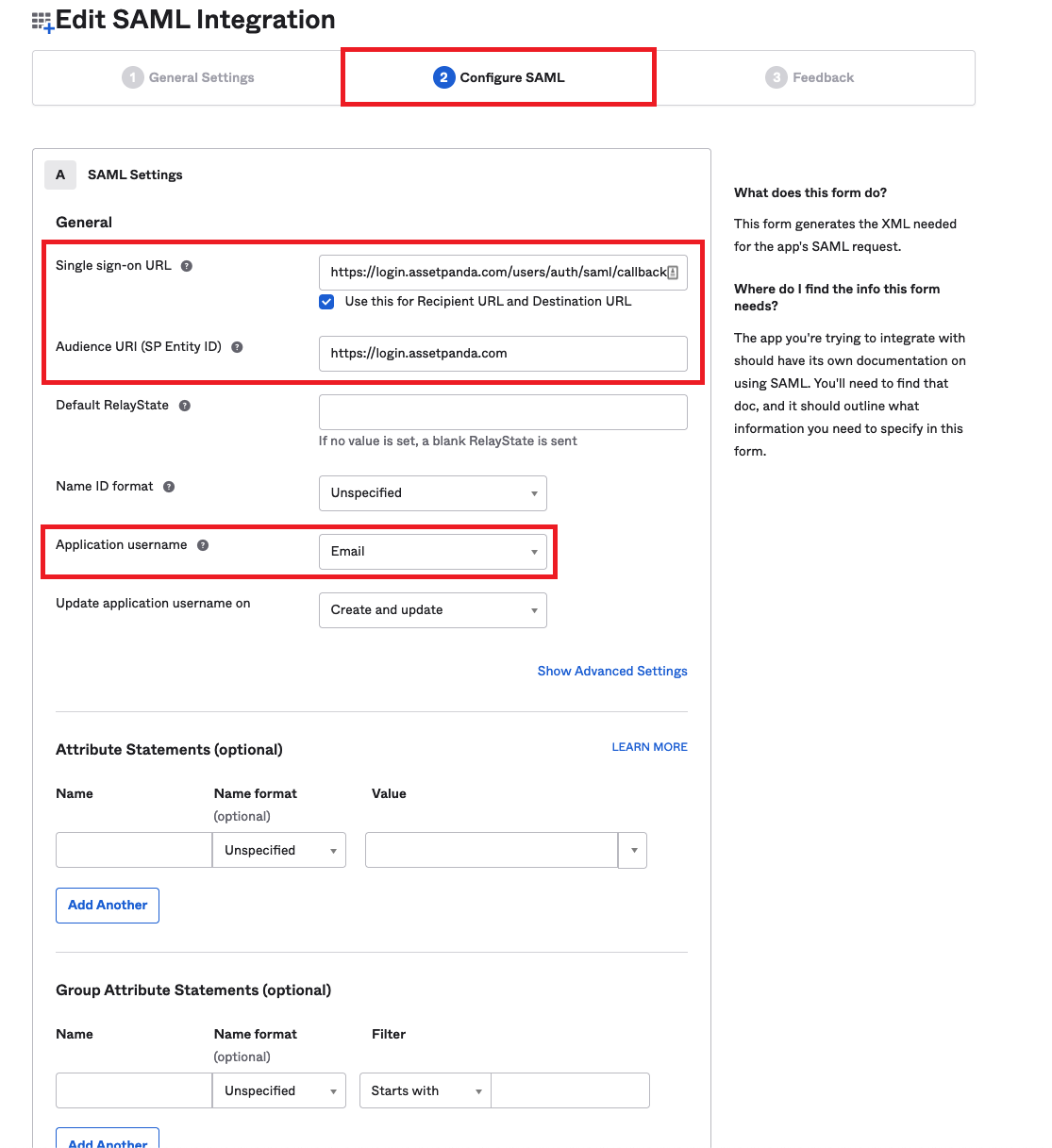A detailed screenshot showcasing the "Configure SAML" integration process on a web application, highlighting the second tab of a three-part configuration sequence. The navigation steps include "General Settings" as the first tab and "Feedback" as the third. This specific section focuses on entering various crucial details for SAML integration. Key input fields are distinctly marked in red boxes, indicating essential information that needs to be filled out. These fields include "Single Sign-On URL," "Audience URI," and "Application Username."

Underneath these primary fields, the form also contains additional optional sections such as "Default Relay State," "Name ID Format," "Application Username," and settings for updating the application username. Further down, optional "Attribute Statements" and "Group Attribute Statements" can be configured if necessary.

To the right, a helpful sidebar provides guidance for users. The section titled "What does this form do?" explains that the form generates the XML required for the app's SAML request. Another section addresses "Where do I find this info?" and advises users to refer to the documentation provided by the application they are integrating with, ensuring they gather all the necessary data to complete the form effectively.

Overall, the image depicts an individual in the process of meticulously inputting the required configurations to successfully integrate SAML, relying on provided instructions to ensure accuracy.